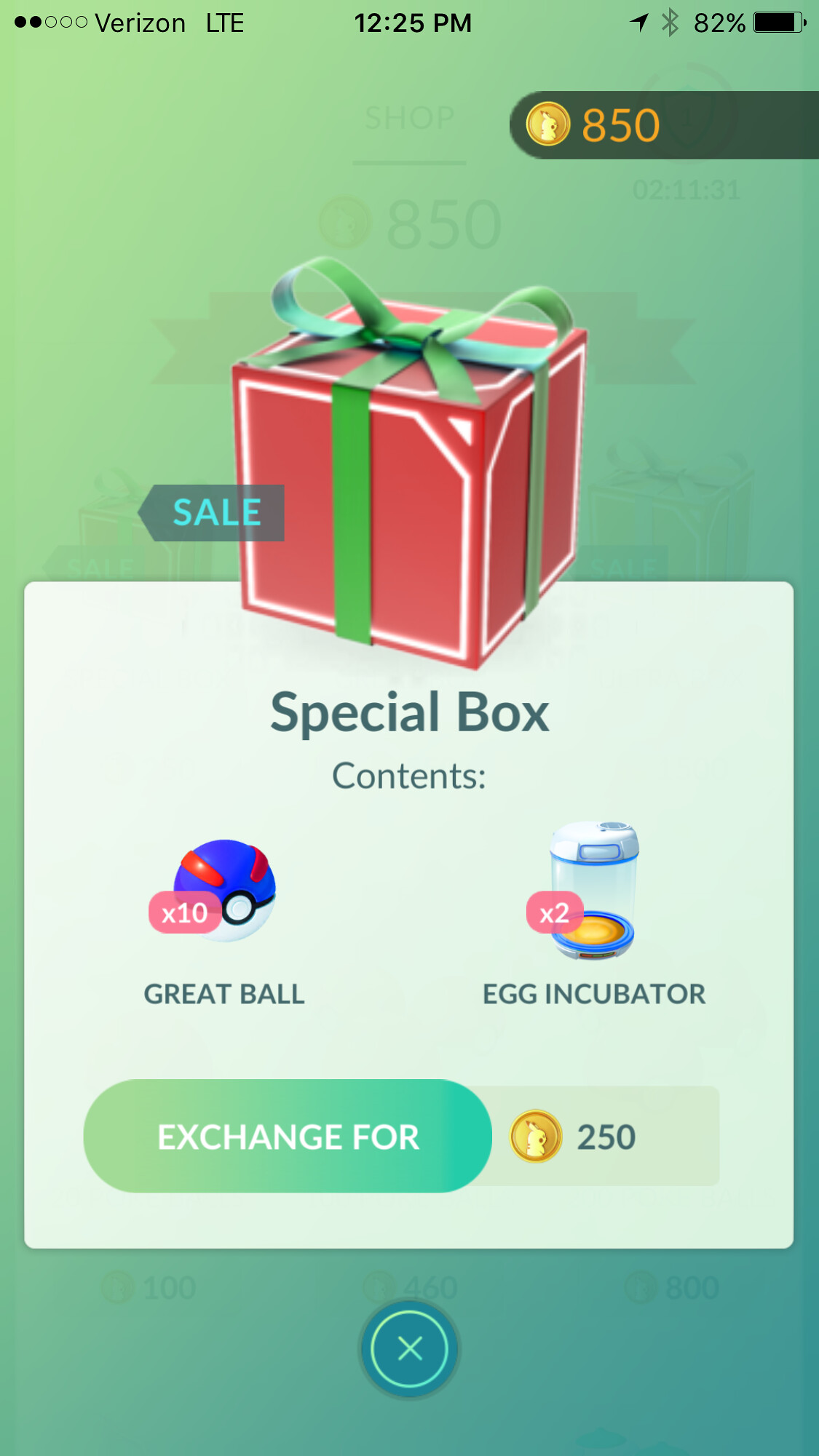The image is a detailed screenshot from a smartphone displaying the mobile game Pokémon Go. At the top of the screen, the status bar indicates Verizon LTE network, the time as 12:25 PM, and an 82% battery charge. The user has 850 in-game golden coins, shown on the upper right corner.

The main focus of the image is a promotional in-game offer. It features a pink loot box with a green ribbon labeled "Sale." Below it, a white box explains the contents: "Special Box" containing "10× Great Ball" and "2× Egg Incubator," each illustrated with their respective images—Pokéballs and incubators with quantity labels. At the bottom of this section, there's a button stating "Exchange for 250" next to a gold coin. The screen background transitions from an aqua hue on the top to a turquoise at the bottom, blending seamlessly. There is an X button at the lower part of the screen to close the window.